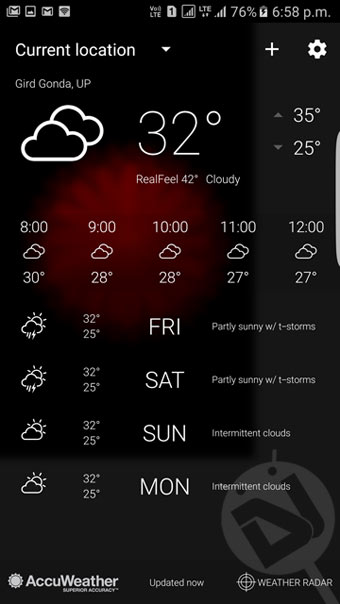The image depicts a smartphone weather application interface, providing a comprehensive view of current and upcoming weather conditions. In the top left-hand corner, messaging and email icons are displayed, indicating the phone's communication tools. At the top right-hand corner, the time is shown as 6:58 PM, with a battery icon at 76%, signal strength indicated by three bars, and a small lightning bolt symbol.

The current location is labeled as "Gerd Gonda," displayed prominently in white text with a downward-pointing arrow, suggesting a dropdown for location settings. Adjacent to this, there is a plus sign and a settings icon for additional options. Below this header, cloud icons and a temperature reading of 32 degrees stand out, with high and low temperatures marked as 35 and 25 degrees respectively, each with an accompanying arrow.

The app further details the weather as "Feels like 42 degrees and cloudy." Following this, an hourly forecast lists the conditions from 8 PM to 12 AM, showing consistent temperatures and cloudy skies: 30 degrees at 8 PM, 28 degrees at 9 PM, 28 degrees at 10 PM, 27 degrees at 11 PM, and 27 degrees at 12 AM.

Towards the bottom, a weekly forecast from Friday to Monday is present: 
- Friday: Partly sunny with thunderstorms.
- Saturday: Partly sunny with thunderstorms.
- Sunday: Intermittent clouds.
- Monday: Intermittent clouds.

AccuWeather is identified as the source at the bottom of the app, with a note indicating it was "Updated now." To the right, a "Weather Radar" link is available.